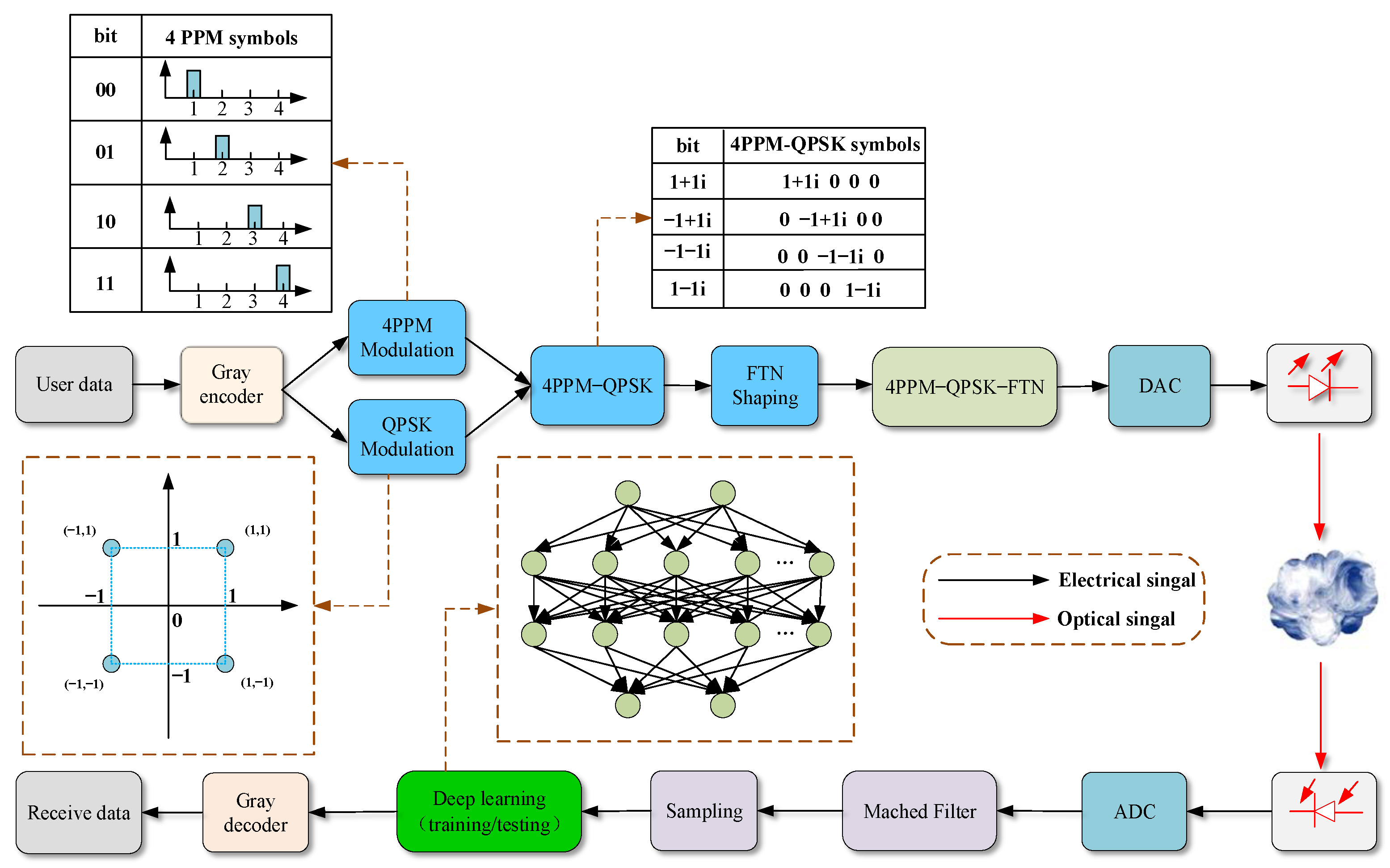The image is a detailed flowchart on a white background illustrating a comprehensive data transmission and modulation process. The diagram contains various colored boxes, each representing a different stage in the signal processing chain. 

Starting in the top left corner, a table lists 'BIT' values (00, 01, 10, 11) alongside corresponding '4 PPM symbols', with graphical arrows pointing up and across. Below this table, additional boxes and tables are arranged horizontally and vertically, linking the various stages of signal modification and data processing.

The stages include: 
- 'User Data' in gray,
- 'Gray Encoder' in pale color,
- '4 PPM Modulation' and 'QPSK Modulation' in blue,
- '4 PPM QPSK FTN Shaping' in blue, 
- '4 PPM QPSK FTN DAC' in olive,
- 'ADC' in blue,
- 'Matched Filter' and 'Sampling' in light purple,
- 'Deep Learning (Training/Testing)' in bright green,
- 'Gray Decoder' in pale peach,
- 'Received Data' in gray.

Different types of signals are illustrated using colored arrows, with blue arrows indicating electrical signals and red arrows indicating optical signals. The stages are connected by these arrows, showcasing the flow from encoding to modulation, signal shaping, and eventual decoding.

Dotted lines encircle specific sections of the diagram, highlighting areas such as clusters of circles and sections featuring arrows for electrical and optical signals. Additional schematic diagrams within the flowchart include a square formed by four circles, a cluster of green circles with intersecting arrows, and an illustration resembling a crystal.

This visually detailed chart clearly outlines the processes involved in signal transmission and modulation, making it a comprehensive reference for understanding data encoding, modulation techniques, and signal processing.